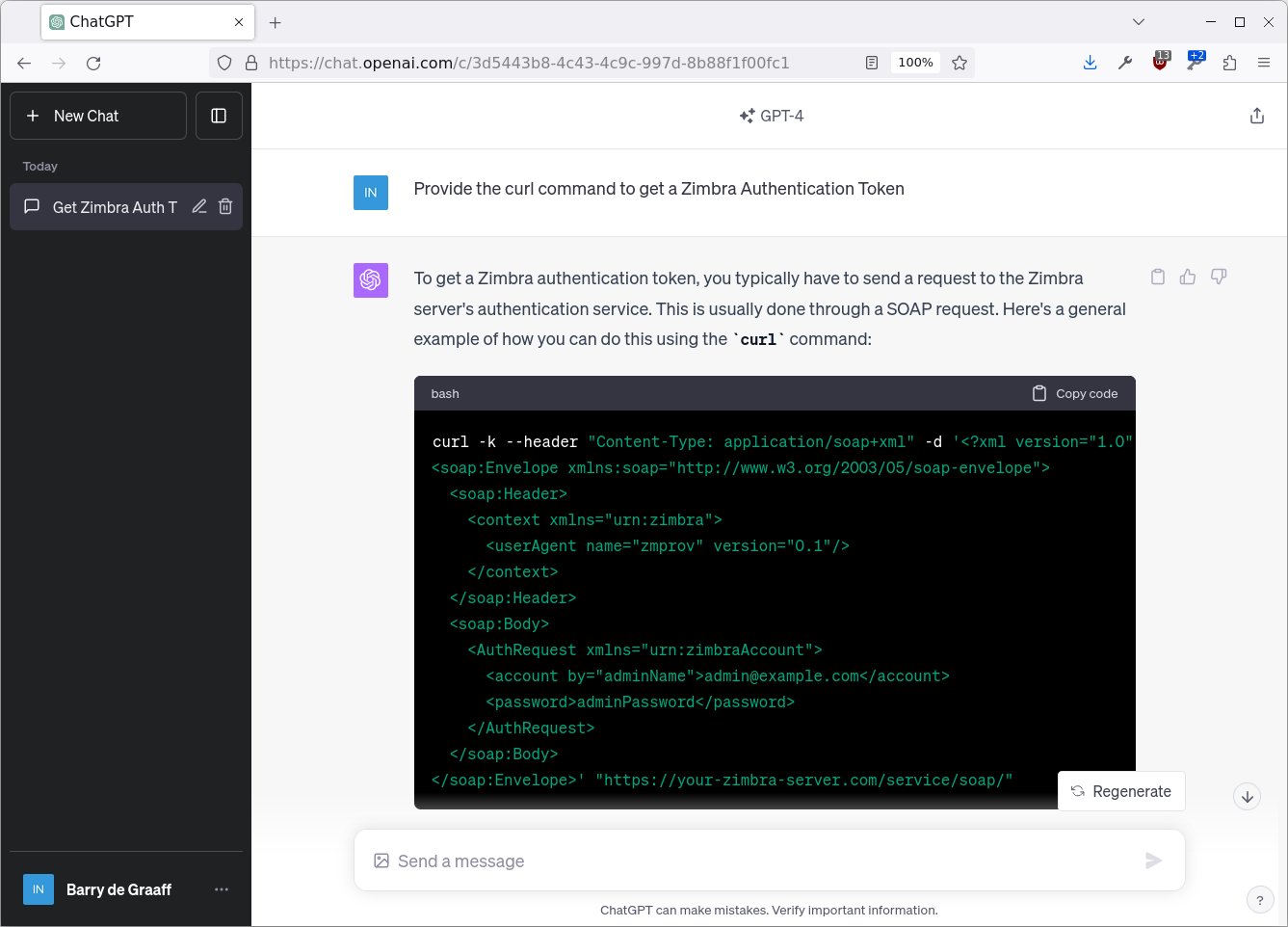**Detailed Caption:**

This image is a screenshot of the AI platform ChatGPT-4 interface. The left side of the screenshot displays a black border with several user interface elements, including a "New Chat" button, a copy icon, and a timestamp labeled "Today." Directly below these elements are various icons: a chat icon with the label "Get Zimbra off," a trash can icon, and an edit (pen) icon. At the very bottom left is an "IN" icon enclosed within a blue square.

In the main body section of the screenshot, a user query is presented asking about obtaining a Zimbra authentication token. The system response explains that to acquire a Zimbra authentication token, one typically needs to send a request to the Zimbra server's authentication service, usually done via a SOAP request. The response further provides an example of how to use the `curl` command for this purpose. Following the provided text, the interface features an input box prompting the user to "Send your message." Finally, a disclaimer at the bottom of the chat emphasizes the importance of verifying critical information, acknowledging that "ChatGPT can make mistakes."

This detailed caption outlines the various interface elements and provides a comprehensive overview of the conversation's content and context within the ChatGPT-4 environment.